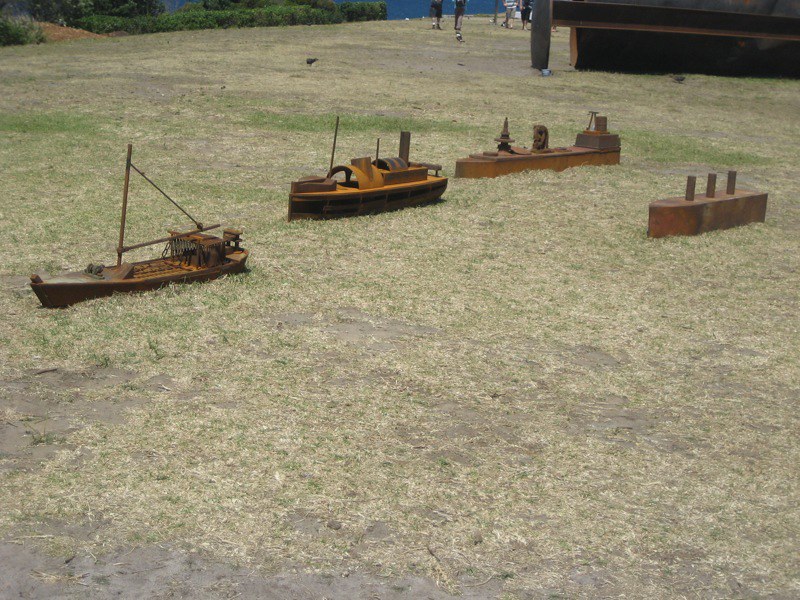This vibrant color photograph captures a meticulously arranged yard decoration featuring four distinct wooden boats set on a sprawling field of freshly mowed grass. The grass, which takes up the majority of the image, appears predominantly white and withered, with scattered patches of green peeking through behind the boats. The boats are aligned in an almost straight, slightly curved line near the center of the image. 

In the background, there’s a blue wall and a large dark brown wooden structure, possibly forming part of the landscape's edge. Additionally, a walkway and shrubbery are visible towards the upper left, enhancing the scene's natural elements. The upper portion of the photograph includes glimpses of people’s feet, suggesting that this might be part of a public display, possibly at a museum or park.

The wooden boats each exhibit unique characteristics. On the far left is a sailboat frame, absent its sail, showcasing just its skeletal structure. Next is a boat resembling a steam-powered vessel with vertical protruding poles, possibly serving as chimneys. The third vessel appears to be akin to a nuclear-powered battleship, also featuring a structure reminiscent of a chimney. Lastly, to the far right is a boat that resembles a trash barge, notable for its three smokestacks. The boats, seemingly floating atop the grass, create a whimsical and artistic scene, blending nautical themes with terrestrial settings.